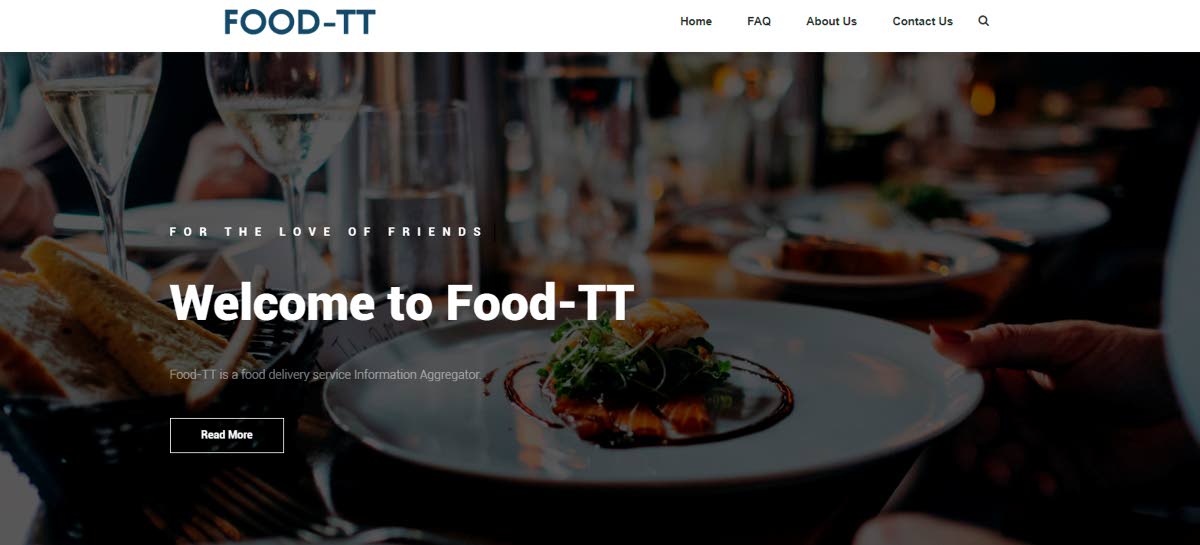The image appears to be a screenshot from a website. In the top left corner, navigation links are labeled "Food-TT," "Home," "Back," "About Us," "Contact Us," and "Vent Fan." The website seems to have a fourth-level category labeled "Friends" and a welcoming message: "Welcome to Food-TT." Food-TT is described as a food delivery service.

The bottom right of the image includes options such as "Read More," "Bread," a pair of glasses, a glass of water, and an elaborate dish. The dish is placed on a table, consisting of salmon garnished with a red sauce spread around it and assorted vegetables. There is also a slice of some kind of fried fish on top. In the background, additional foods, dishes, plates, glasses, and tables are visible.

A person with red nail polish is seen in the scene, and there is a basket of bread nearby. The repetitive navigation labels "Home," "Back," "About Us," and "Contact Us" suggest possible website elements or navigation aids. Another prominent dish near the person appears to be skillfully prepared, adding to the abundance of food and dining elements present.